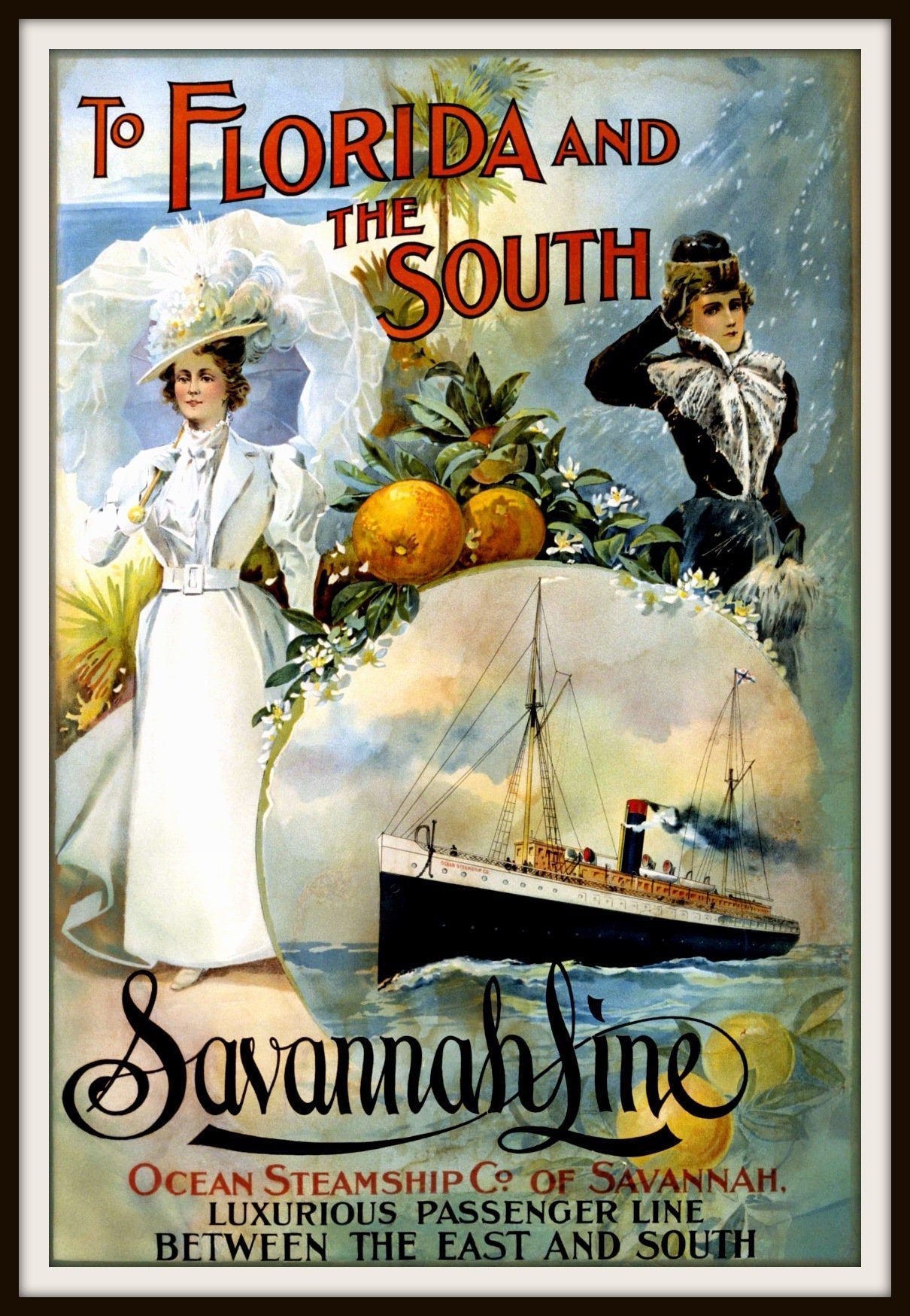The image depicts a vintage poster, likely from the late 1920s, advertising the Savannah Line of the Ocean Steamship Company of Savannah. The main text, in striking red letters, reads "To Florida and the South." The central figure is a woman in an ornate, old-fashioned white dress adorned with lace and silk, paired with a wide-brimmed hat decorated with flowers. To the right, another woman appears, dressed in a form-fitting black outfit with fur lapels and a fur cap, raising her hand in a salute. A steamship is pictured on the water, enhancing the historic and luxurious feel of the scene. At the bottom of the poster, "Savannah Line, Ocean Steamship Company of Savannah" is elegantly inscribed, suggesting prestigious travel routes between the East and South. The artwork is framed, bordered in black with a white trim, adding to its presentation as a beautiful, artistic piece ideal for display.